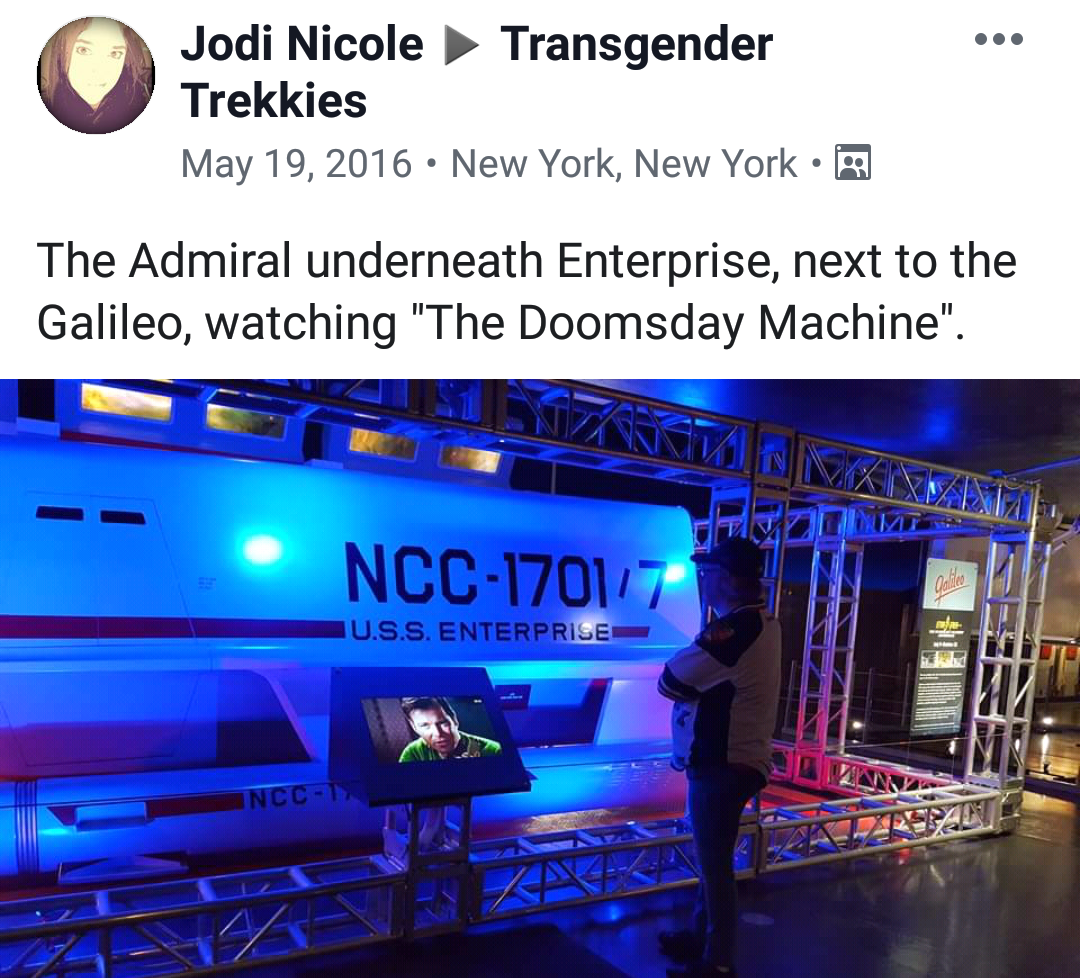This image features a social media post advertising a public event showcasing a Star Trek exhibit. At the top, there's a circular avatar of a woman with brown hair, accompanied by bold black text that reads "Jodi and Nicole Transgender Trekkies." Below this, in smaller gray print, the date "May 19th, 2016, New York, New York" is displayed. A headline follows in slightly larger font: "The Admiral underneath Enterprise next to the Galileo watching 'The Doomsday Machine.'" 

The main body of the post includes a horizontal, rectangular photograph of a Starfleet shuttlecraft, labeled "NCC-1701/7, USS Enterprise," with blue piping along its edges. The shuttlecraft, believed to be from the Star Trek TV episodes, is encased by a metal framework designed to prevent touching. In front of the display, there's a podium featuring a still of James Kirk, portrayed by William Shatner. A man dressed in a blue and white t-shirt, jeans, and a trucker hat is seen standing before the exhibit, intently observing it. The background of the social media post is a simple, clean white, making the details of the event and exhibit stand out prominently.